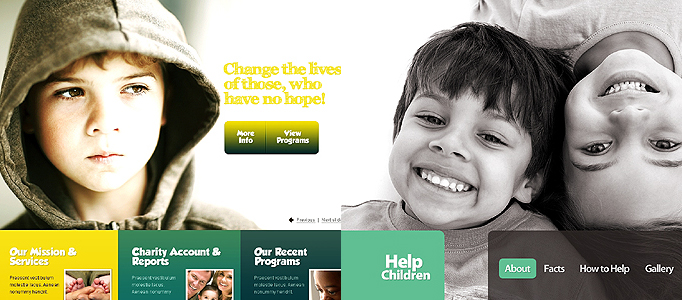On the left side of the image, a color photograph features a boy wearing a gray hood. Adjacent to it on the right side, there is a black-and-white photo of two children: one lying face-up and the other face-down. Bright yellow text, which is difficult to decipher, appears between them. 

Above these images, a yellow rectangle transitions to a dark green shade and contains the text, "More Info." Below it, a line separates the sections with labels "View Programs" and "Help Children." 

To the left, another yellow rectangle has white text that is too small to read, accompanied by an image at the bottom resembling feet. Next, a green rectangle labeled "Charity Account and Reports" includes pictures of faces and additional small text. 

There is also a blue rectangle titled "Our Recent Programs," containing more unreadable text and an image displaying a person's face. Following this, a light green rectangle is labeled "Help Children."

Further down, a gray rectangle encloses a light green box labeled "About," alongside the titles "Facts," "How to Help," and "Gallery."